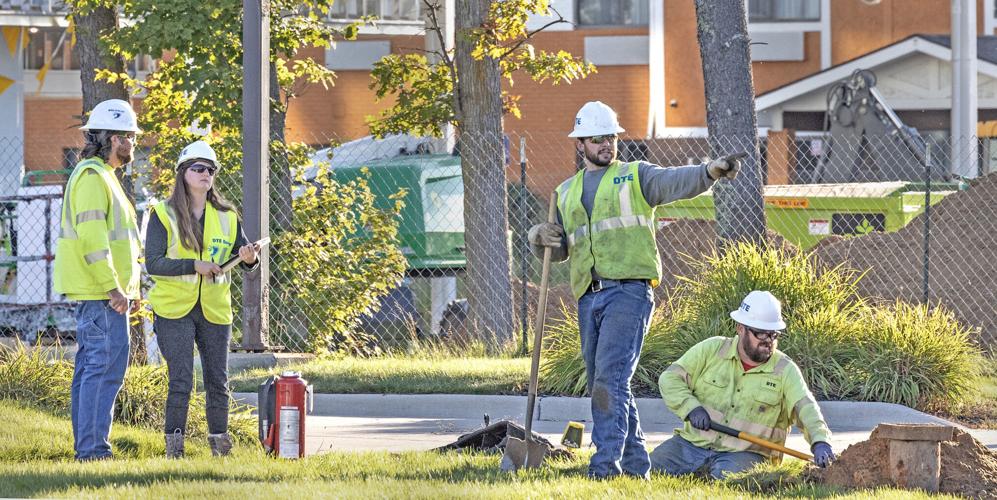This detailed color photograph captures a vibrant outdoor construction scene on a sunny day. Four construction workers, distinguished by their safety attire, are prominently featured in the foreground. Each worker dons a fluorescent yellow-green safety vest adorned with the logo and green print "DYE," along with white helmets marked with a blue logo. Additionally, three of the workers sport blue jeans, while the female worker, who has long brown hair, opts for black jeans. All workers are equipped with sunglasses, except for one, making it harder to discern if he also wears any.

The workers are split into two groups: to the left stand a man with long graying hair and a woman, both gazing into the distance. On the right, two men are engaged more actively with the task at hand; one of them is seated within a dug hole, while the other stands holding a shovel and gesturing.

The scene is set against a grassy area with a concrete roadway directly behind the workers. Adjacent to the construction team, a red fire extinguisher is visible. The background reveals a chain-link fence, beyond which a red-orange brick building with white-trimmed windows stands, partially obscured by tree trunks and foliage, some leaves turning from green to yellow. Additionally, construction equipment is visible in front of the building, contributing to the dynamic industrial ambiance.